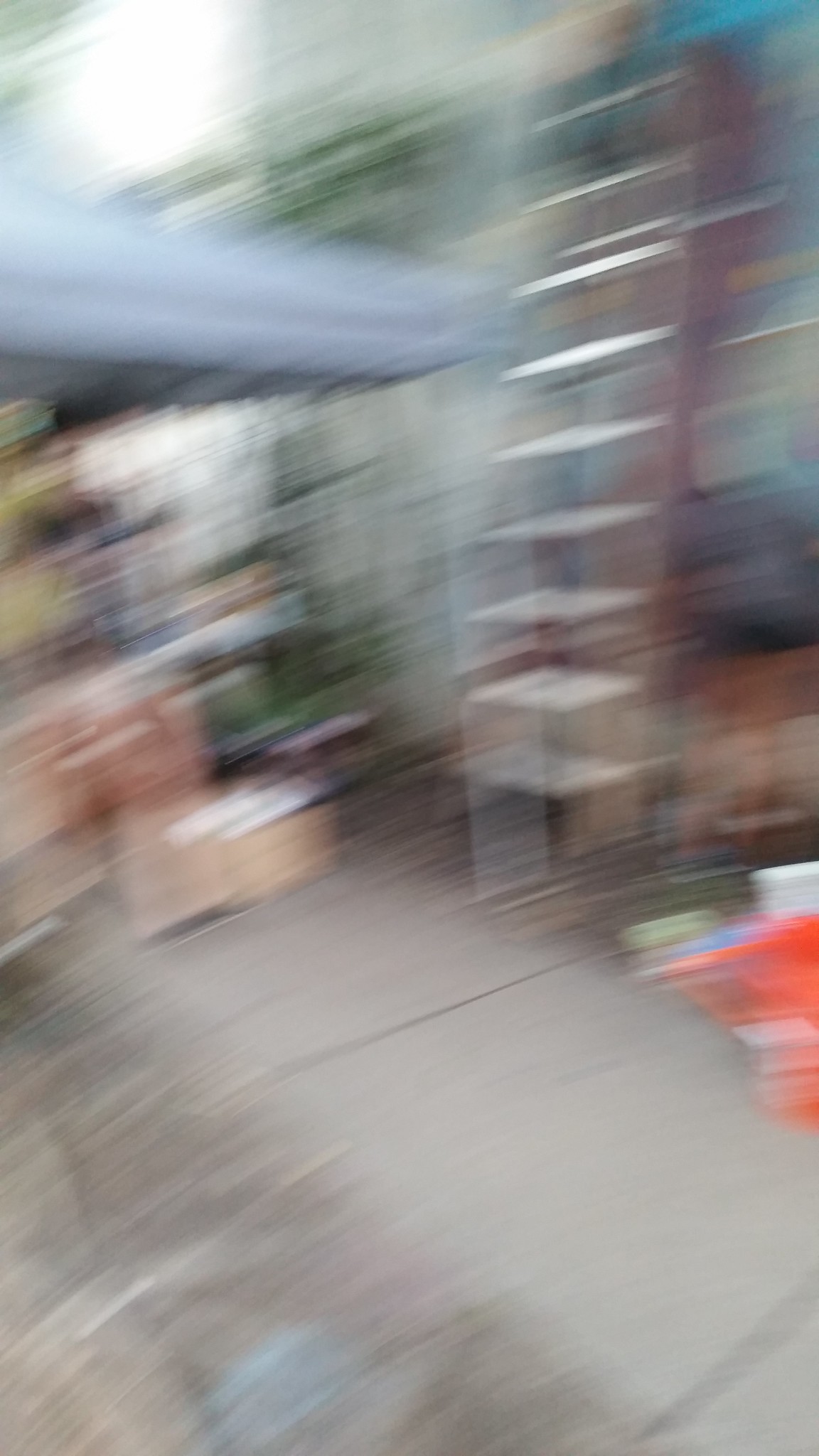This photograph, taken outdoors, is extremely blurred with notable motion blur. The image predominantly features a gray concrete walkway with visible expansion joints, starting from the bottom right corner and extending towards the center left. To the end of the walkway, there appear to be several stacked brown boxes. In the lower and upper left corners, the edge of a structure, possibly a gazebo or an opened garage door painted in dark gray or faded blue, is visible. On the right side, near the concrete path, there's a bright orange blur, which seems to be objects like buckets with some white and green elements. Just above this, there is an empty tall metal rack or shelving unit, with distinct horizontal and vertical lines suggesting shelves and supports, possibly a ladder. Behind this rack, there is a wall. Additionally, the upper left corner of the image shows some light reflections, hinting at fluorescent lights turned on in the background. Scattered across the concrete floor are indistinct objects, including what might be cement bricks and items colored bright orange-red. This setting could be an outdoor area near a garage or basement-like environment.